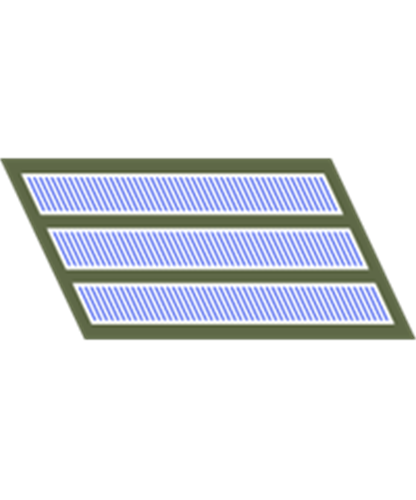The image illustrates a dark gray metallic ceiling vent cover with a parallelogram shape, designed for air filtration in home or office duct systems. The vent has two horizontal stripes across its border and a series of louvers in between that allow air to pass through. These louvers, in various shades of gray, are accompanied by three white vertical panels with blue diagonal lines, evoking a sense of reflection, similar to thin-style windows from the previous World Trade Center site. The vent cover, which blends seamlessly with the surrounding ceiling, ensures that air entering the ducts is filtered, thus reducing the need for frequent duct cleaning. The entire frame is set against a white background, highlighting its utilitarian design and minimalistic aesthetics.